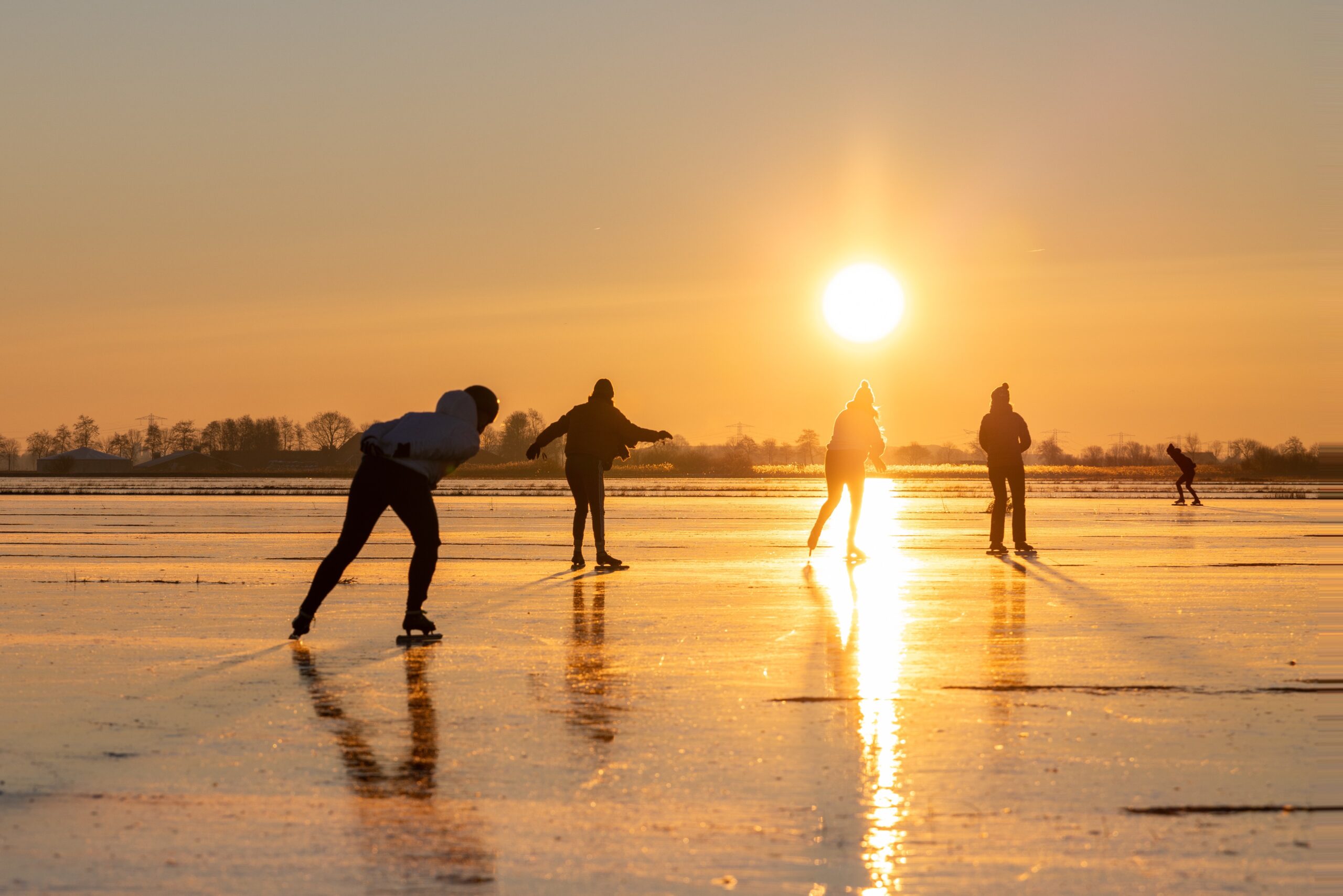The image depicts a serene scene of five people ice skating on a frozen lake during either sunrise or sunset, as the bright golden sun casts a hazy glow across the sky. The sun, slightly to the right and near the center of the photograph, illuminates the silhouettes of the skaters who are wearing a mix of helmets, hats, and coats. Most of them are in motion, skating towards the direction of the sun, with the ice surface appearing slightly rough. The a tree-lined far background includes some telephone poles, electrical wires, and farm-like buildings, contributing to the tranquil, peaceful ambiance of the scene.